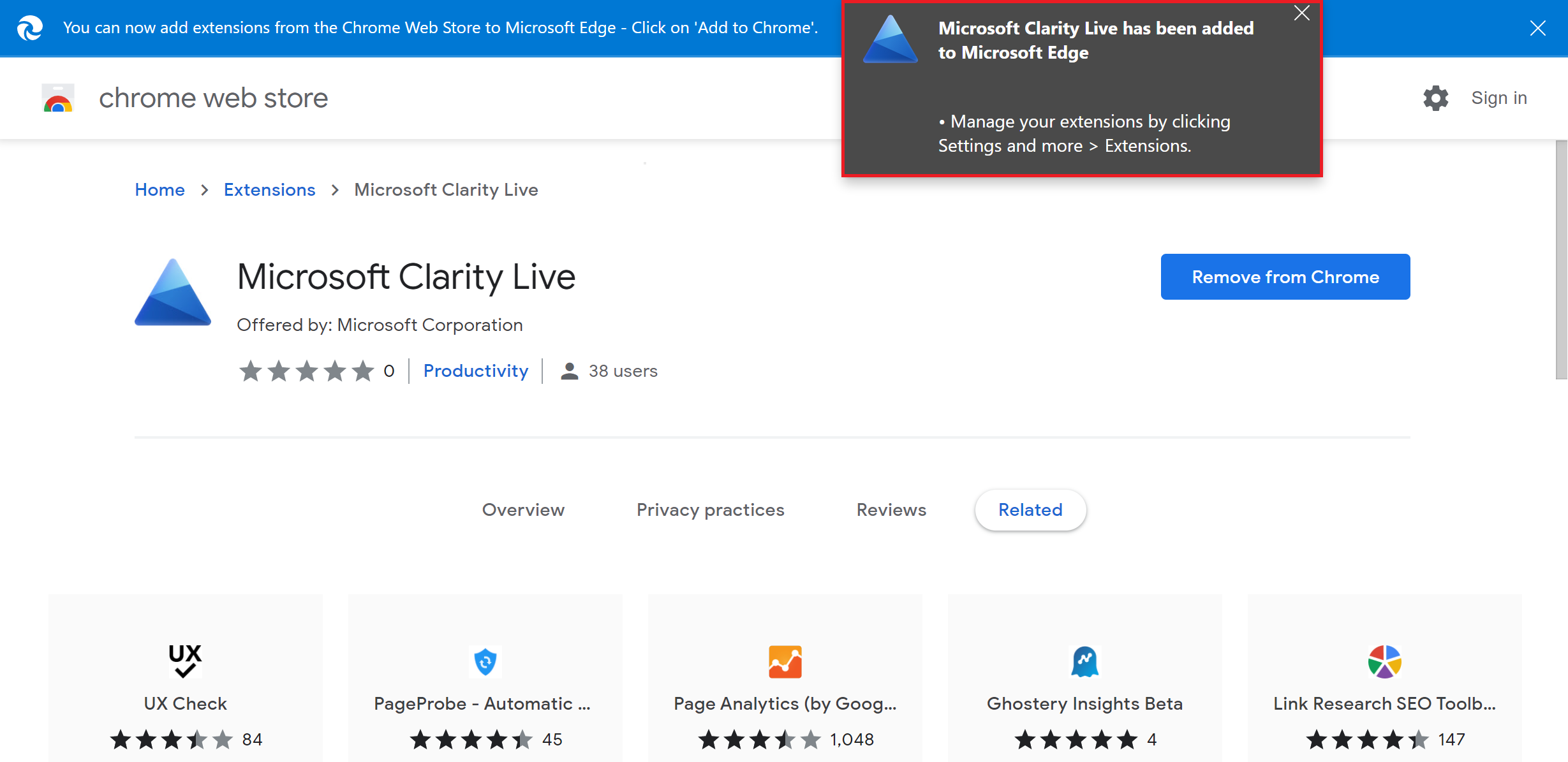**Detailed Caption:**

The image is a screenshot of the Chrome Web Store, displayed in a browser with a predominantly white background. At the top of the screen, there is a prominent blue bar with text indicating that extensions from the Chrome Web Store can be added to Microsoft Edge. The text suggests clicking on "Add to Chrome" to proceed. 

Below this, a gray pop-up box with a red outline is visible. It features a blue, three-tone triangle icon in the upper left corner which indicates a notification that reads, "Microsoft Clarity Live has been added to Microsoft Edge. Manage your extensions by clicking settings and more extensions." 

Further down the screen, on the left side, there is the Chrome logo next to the words "Chrome Web Store," accompanied by the blue triangle icon and the text "Microsoft Clarity Live," which is offered by Microsoft Corporation. This section also mentions that the extension falls under the "Productivity" category and includes a star rating for the extension. 

To the right of these details, there is a large, clickable blue rectangle that says "Remove from Chrome," indicating an option to remove the extension.

At the bottom of the screen, as part of the "Related" section, there are five gray squares with different symbols and names of other extensions. The first square features a "UX Check" extension with a rating of approximately three and a half stars and the number 84. Another square displays an icon resembling a blue ghost for the "Ghostory Insights Beta" extension, rated at five stars. Several other related extensions are also displayed in this section.